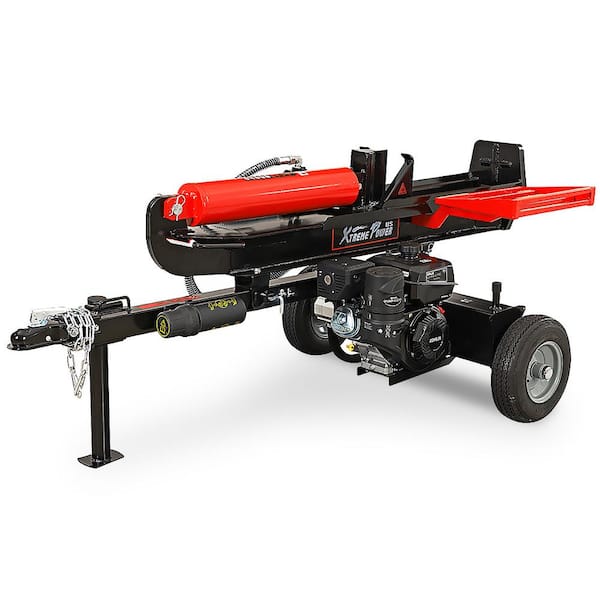This image depicts a horizontally-oriented, towable piece of equipment designed for transportation via its attached trailer hitch. The machine boasts a sleek black body accented with striking red components, including a red platform and a cylindrical gas motor positioned beneath. The red platform likely facilitates boarding or accessing the machine. A chain is attached to the tow hitch, ready to be connected to a truck or SUV for mobility. Notably, visible text on the side reads "Extreme Power," hinting at the equipment's functionality, possibly as a high-powered log splitter driven by a pneumatic or hydraulic cylinder. Set against a plain white background, the machine rests quietly, unhitched and stationary, showcasing its sturdy construction and modern design likely intended for field or work yard use.